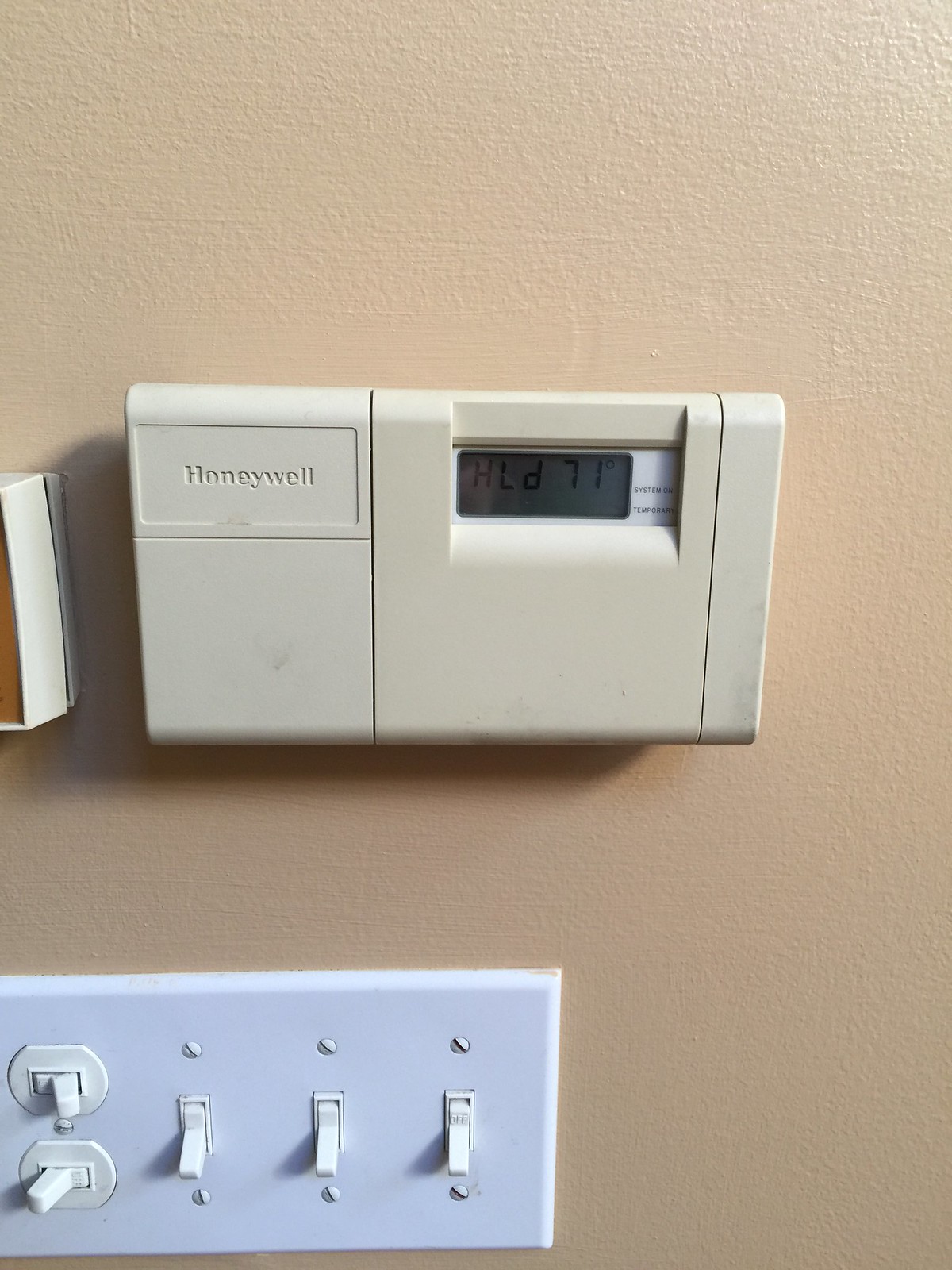The image depicts a wall painted in a soft, pale cream-brown hue. Located towards the bottom left is a white light switch panel featuring five individual switches. Notably, the two switches positioned on the left side of the panel are oriented vertically, requiring a left-to-right motion to operate, unlike the conventional up-and-down orientation. The remaining three switches are aligned in the standard vertical direction, with all currently in the off position except for the topmost switch.

Above the light switch panel is an off-white Honeywell thermostat panel, exhibiting some smudged dirt marks. The thermostat is closed, partially obscuring the buttons. It displays an abbreviated message "HLD" indicating "HOLD," with a temperature reading of 71 degrees Fahrenheit. The panel confirms that the system is on with a clear text readout.

To the left of the Honeywell thermostat, there appears to be another panel, though its purpose is indeterminate from the image. The image primarily focuses on the detailed interplay between the light switch panel and the Honeywell thermostat.